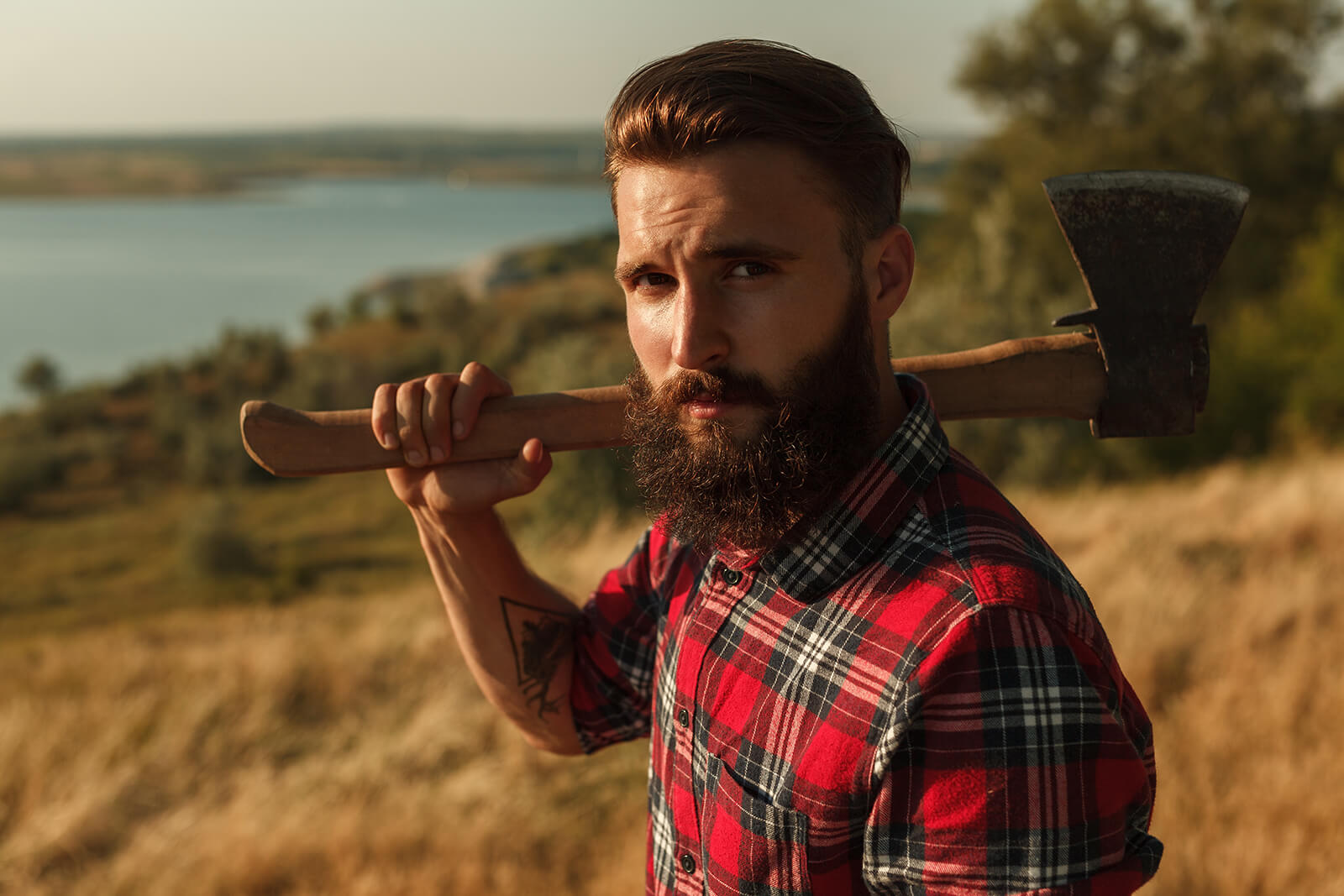In this photograph, the main subject is a handsome young Caucasian man with long auburn hair, which is brushed back and shaved on the sides. Complementing his hair is a matching long, dark brown beard, and mustache. He is holding a hatchet or small axe over his right shoulder, displaying a confident and rugged demeanor. He wears a brand-new red flannel shirt, rolled up to his biceps, which features a pattern of black and white checkered boxes. A distinctive triangular tattoo adorns his right forearm. The man is standing on a bank of tan-colored grass, gazing directly at the viewer, with the background slightly blurred but revealing a scenic setting. Behind him, green bushes cascade down a hill towards a large river or lake, possibly the Columbia River. The opposite shore is lined with green trees. The photo is captured in late evening light, as evidenced by the soft shadows cast across the man's face, adding to the image's rustic and serene atmosphere.